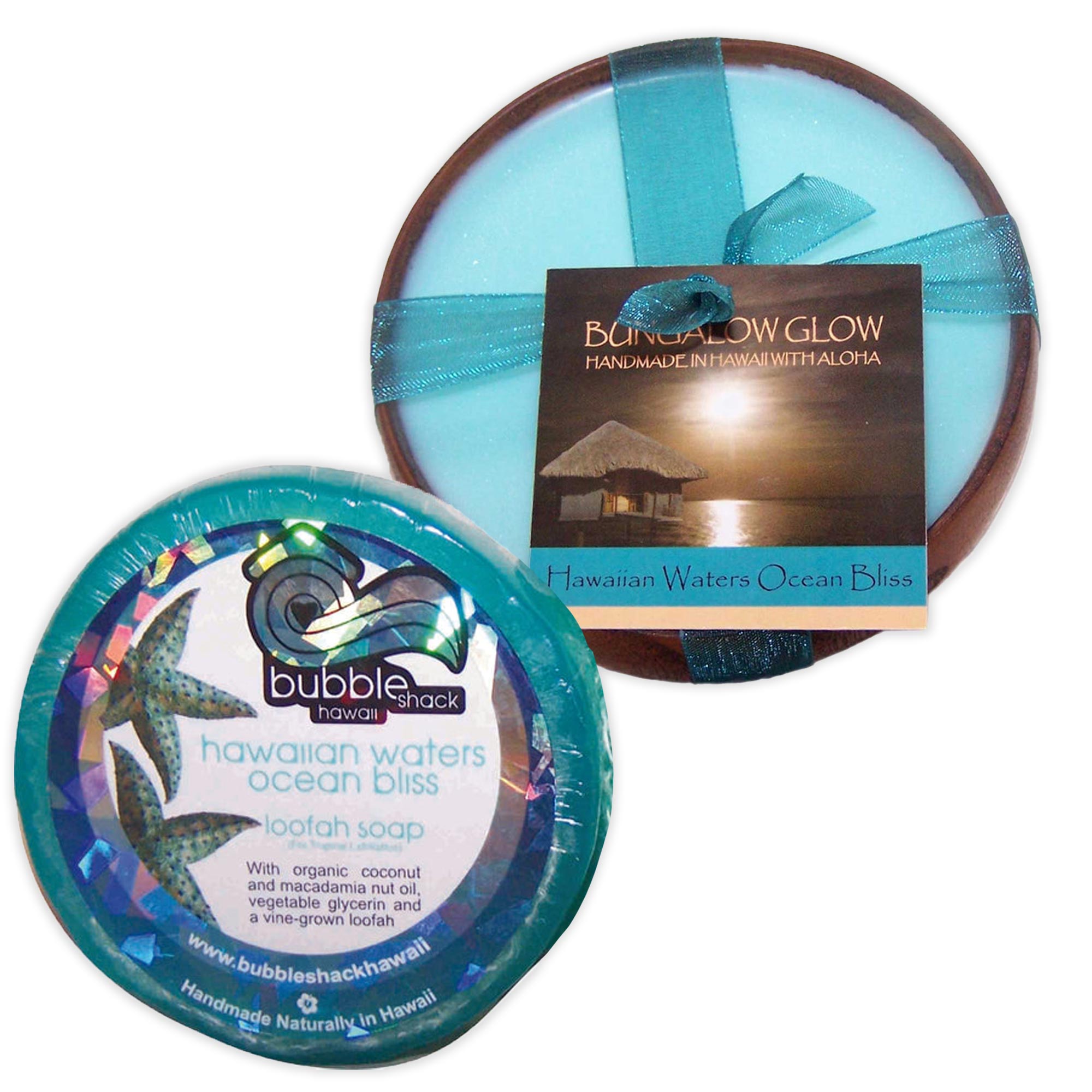The image showcases two round bars of luxurious soap set against a white background. The top soap, encased in a circular wooden rim, is light blue and adorned with a blue bow. It features a label that reads "Bungalow Glow Handmade Hawaiian with Aloe, Hawaiian Waters Ocean Bliss." Below and to the left, a second soap, outside its wooden casing, is wrapped in plastic. This soap bears a detailed label illustrating two starfish and a wave logo containing a black heart. The label reads "Bubble Shack Hawaii, Hawaiian Waters Ocean Bliss Loofah Soap with organic coconut and macadamia nut oil, vegetable glycerin, and vine-grown loofah," followed by the website "www.bubbleshackhawaii.com." Both soaps suggest a high-end, handmade quality reminiscent of products found in specialty boutiques rather than supermarkets. The overall presentation conveys a sense of artisanal craftsmanship and tropical allure.